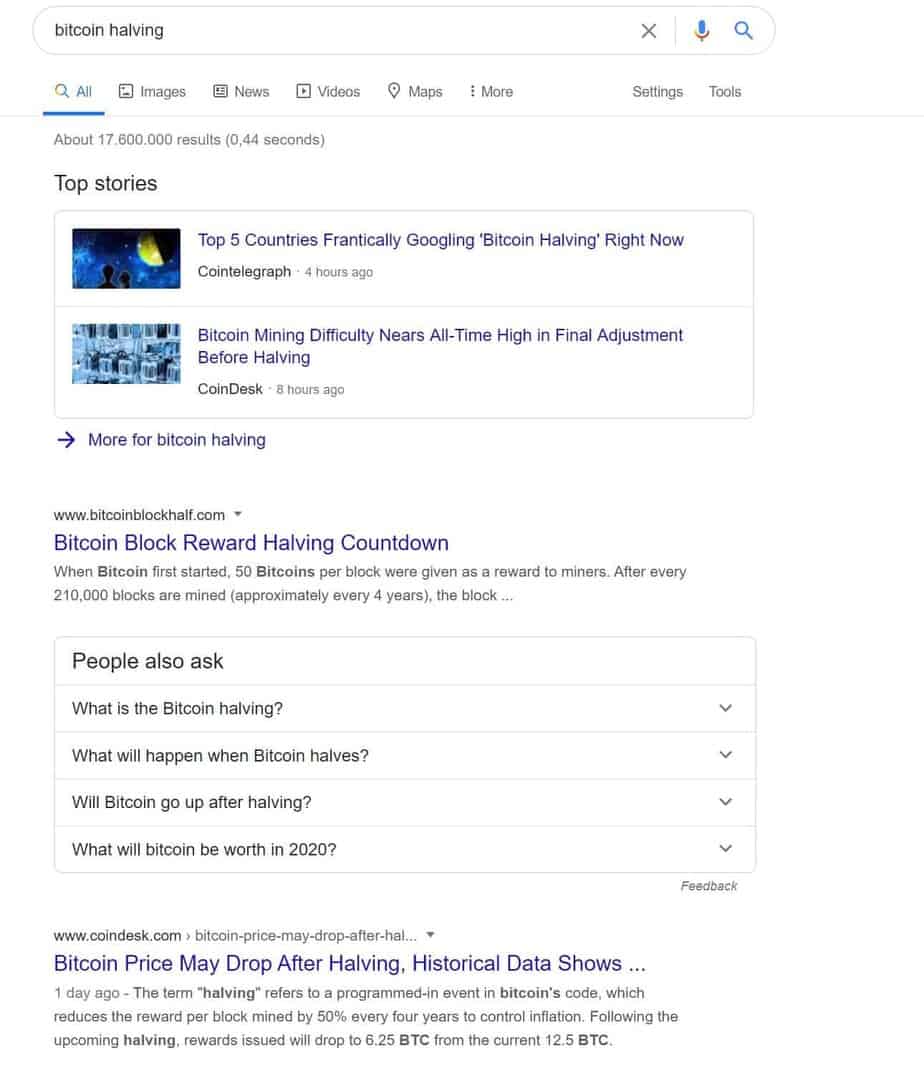A computer screen displays an image of a mobile device screen. The mobile screen has a predominantly white background with numerous words and texts displayed in black and navy blue fonts. At the top of the mobile screen, there is a search bar containing the query "bitcoin halving." Below the search bar, black text reads "Top stories." Further down, the image features two articles. The first article is titled "Top 5 countries practically googling bitcoin halving right now," while the second article reads "Bitcoin mining difficulty nears an all-time high in final adjustments before halving." The image captures a moment focusing on current trends and key updates regarding Bitcoin halving.